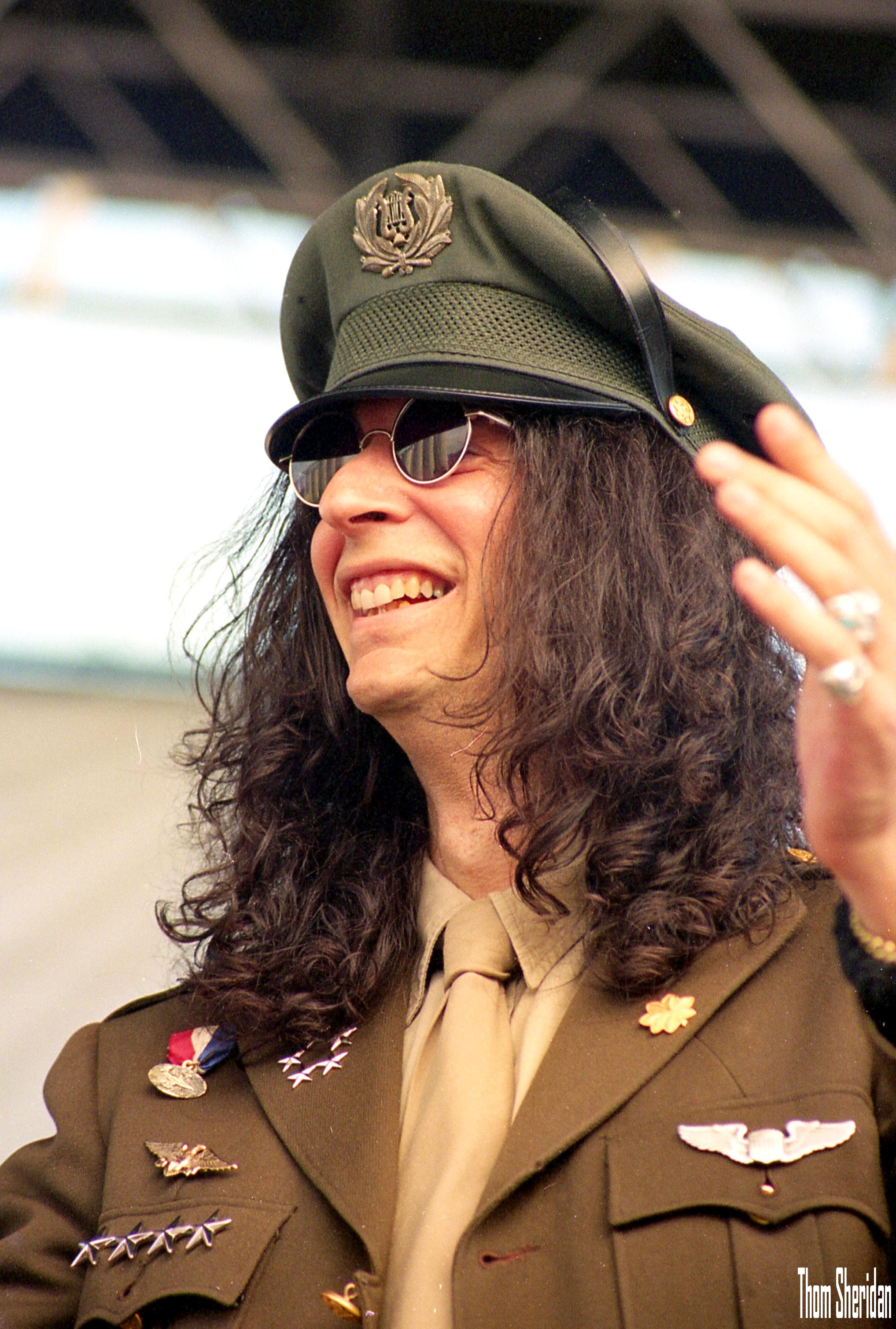This image features Howard Stern, the renowned radio announcer and celebrity, striking a confident pose. He sports his signature long black hair cascading down to his shoulders and is seen wearing dark sunglasses. Stern is dressed in a seemingly military-inspired ensemble, though it appears to be more of a costume rather than an official uniform. 

He dons a green military-style cap with a black bill, adorned with a distinctive emblem at the front. His outfit includes a brown military jacket featuring several notable insignia. On his right shoulder, there's a prominent red, white, and blue medal typically awarded for service, with a set of pilot wings directly beneath it. Below these, the pocket bears the decoration of four stars. On the left side, a matching set of wings is displayed on the pocket, while a star adorns the left lapel.

Stern wears a light brown shirt and matching tie under the jacket, completing the authentic look. His left hand, raised in the air, showcases rings on his fingers, adding a touch of personal flair. Stern’s smile suggests he is enjoying the moment. The background of the image is a blend of light brown and white hues, providing a neutral backdrop that allows Stern's outfit and persona to stand out.